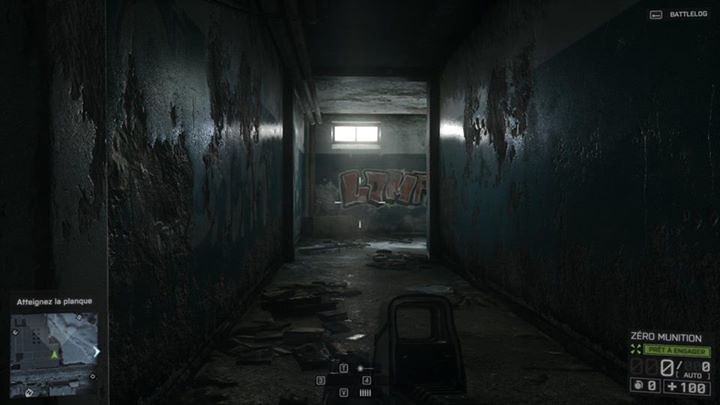This image depicts a highly realistic and immersive scene from a video game, showcasing stunning 4K quality graphics. The player appears to be navigating a dimly-lit, narrow hallway adorned with vibrant graffiti on the far wall. The realism is so profound that it almost blurs the line between a digital environment and a real-world setting. In the bottom right-hand corner of the screen, a HUD element displays "0 munition," indicating that the player has exhausted all their ammunition, suggesting this is a first-person shooter game with survival elements. In the top right-hand corner, small white text reads "Battle Log," likely providing real-time updates or statistics relevant to the game's progress. The bottom left corner contains a smaller screen, possibly functioning as a rearview monitor to enhance situational awareness for the player. Overall, the atmosphere is tense and eerie, encapsulating the player in a thrilling quest for survival and re-supply.